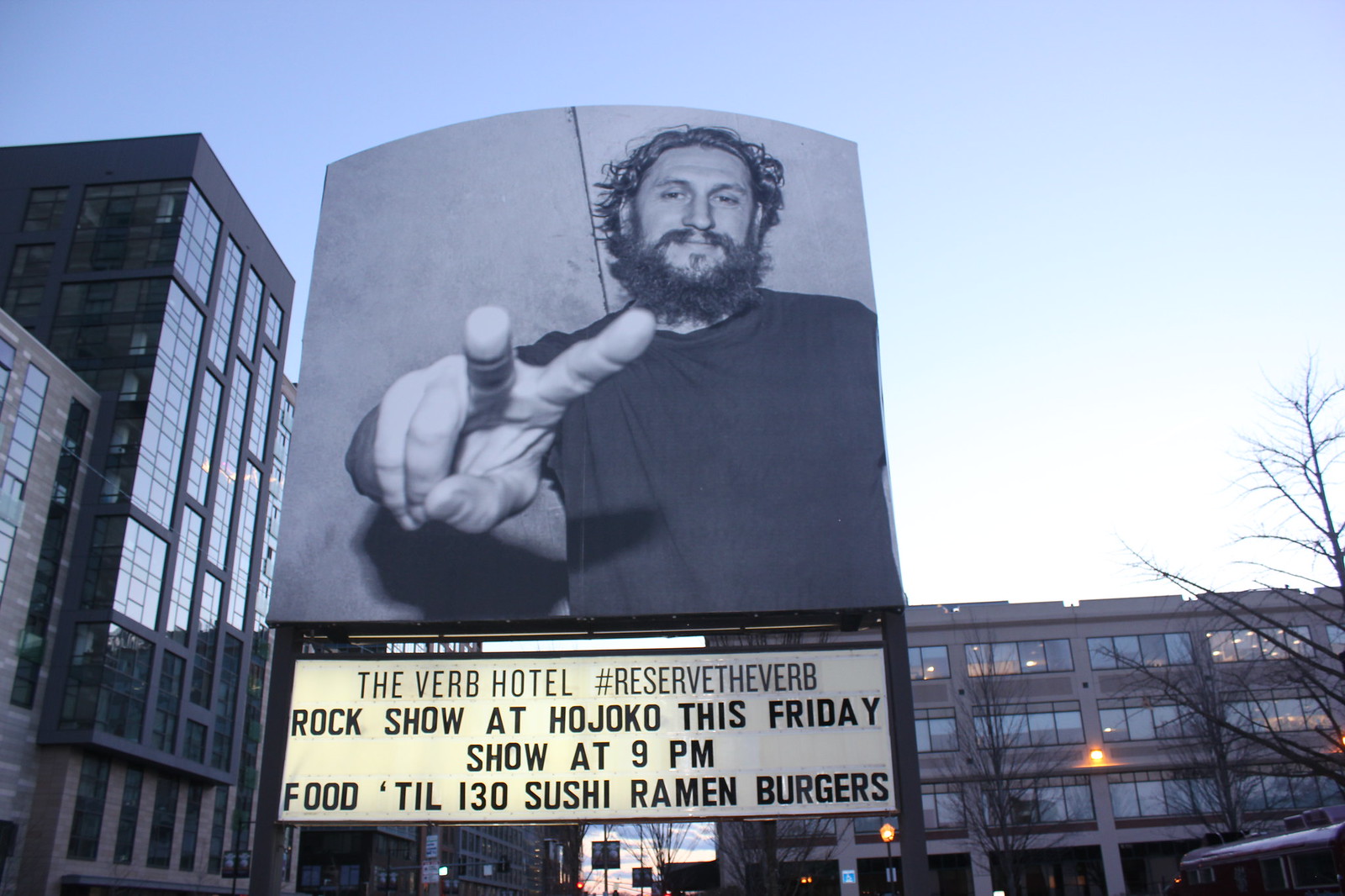The image prominently features a black-and-white billboard situated in front of an impressive, tall building. The billboard displays a large photograph of a bearded man with dark wavy, somewhat long hair, and a mustache, wearing a black sweater or long-sleeved shirt, making a peace sign. Below this photograph is a white, traditional-style marquee with black lettering reading, "The Verve Hotel," followed by "#reservetheverve" and "Rock Show at Hojoko this Friday, show at 9 p.m., food till 1:30." The food offerings include sushi, ramen, and burgers. The scene captures surrounding buildings and a clear blue sky as part of its vibrant urban setting.